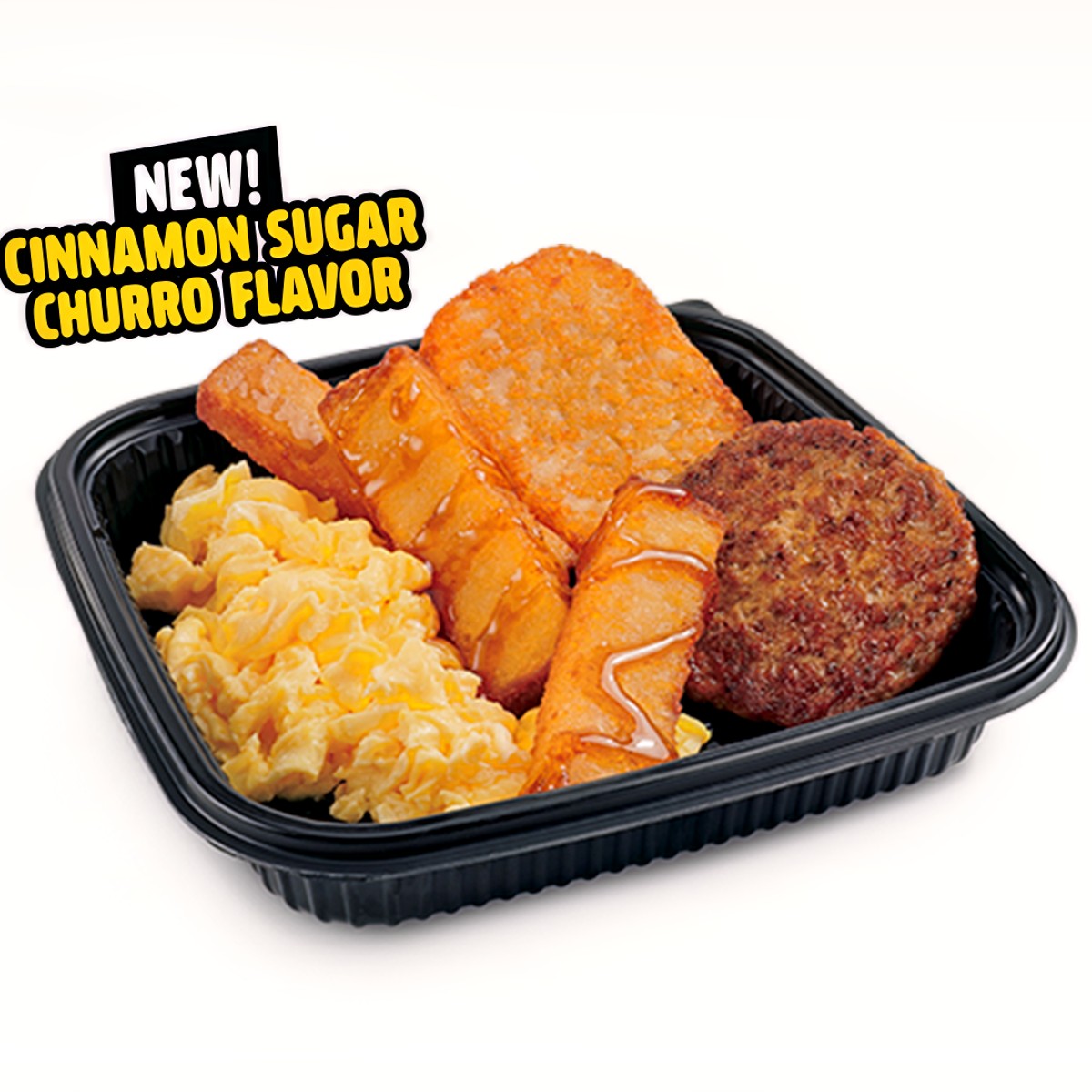This image features a microwavable dinner displayed against a white background. The dish is a black plastic takeout container with ribbed sides and a wider lip than its base. The container is tilted slightly, presenting the food attractively. In the top left corner of the image, a black skewed rectangle with white uppercase text reads “NEW!”, followed by two lines of yellow capitalized text with a black border stating “CINNAMON SUGAR” and “CHURRO FLAVOR.” 

Inside the container, on the left, are yellow scrambled eggs occupying about a third of the dish. Centered are three golden brown French toast sticks drizzled with syrup in a wavy pattern. To the right, there's a flat, golden brown, rectangular hash brown. In the lower right corner is a dark brown, crispy sausage patty. The overall presentation of the food has been slightly propped up to enhance its appeal in the photo.